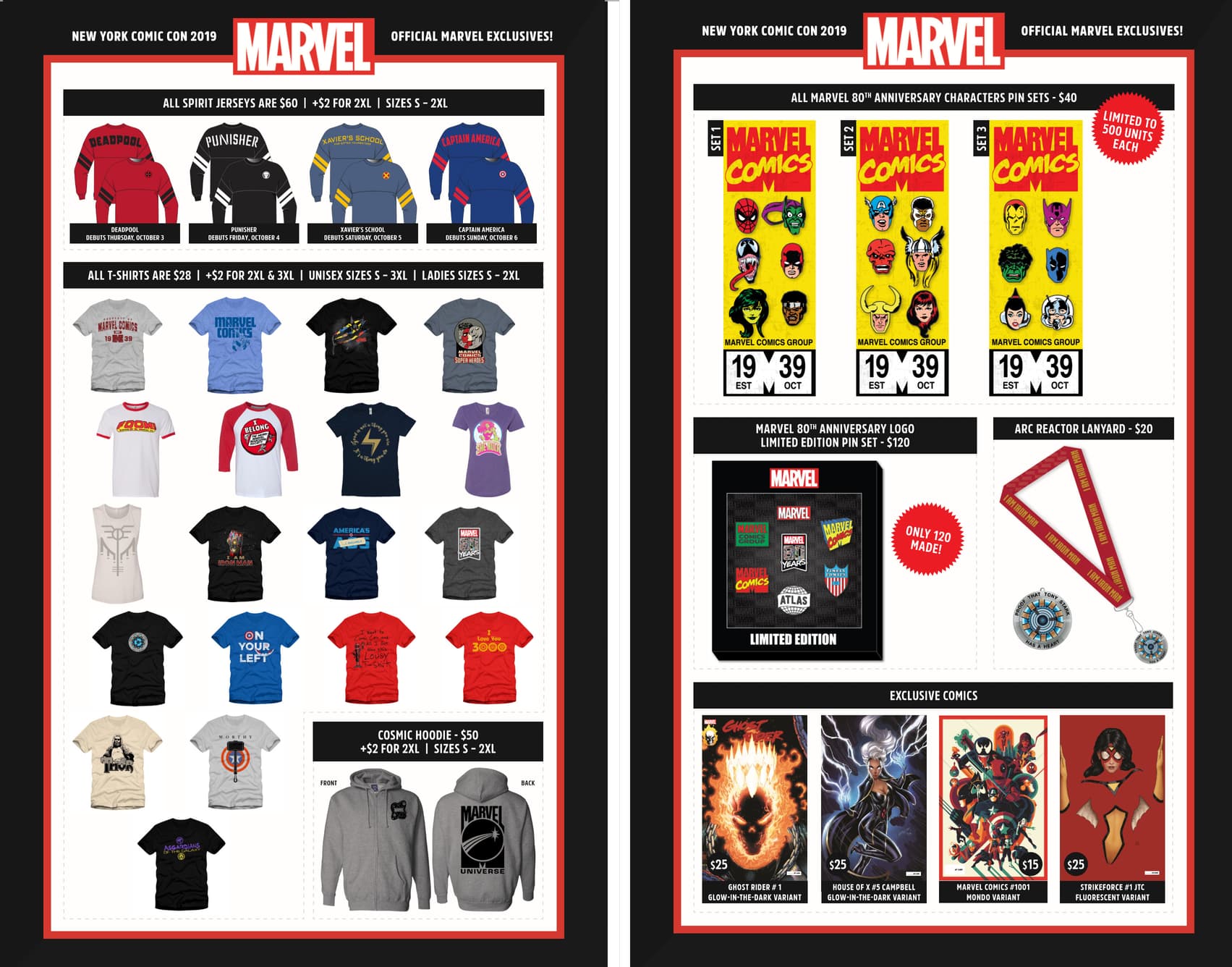This image features two white-on-black posters with a red border from the New York Comic-Con 2019, showcasing Official Marvel Exclusives. The Marvel logo is prominently displayed at the top. Both posters are filled with small images of exclusive merchandise.

The left poster highlights various clothing items available at Comic-Con. At the top, a row of spirit jerseys is priced at $60 each, with an additional $2 for sizes 2XL. The jerseys feature designs for Deadpool, Punisher, Xavier, Skull, and Captain America. Below this, all t-shirts are listed at $28, with an additional $2 for 2XL and 3XL. The unisex sizes range from small to 3XL, while ladies' sizes go from 2 to 2XL. There are 19 different t-shirt designs, each colorful and adorned with various Marvel logos and characters. In the bottom-left corner, a gray front-and-back hoodie labeled "Marvel Universe Cosmic Hoodie" is priced at $50, with an additional $2 for 2XL sizes.

The right poster focuses on collectible items. It features three Marvel 80th anniversary character pin sets, each priced at $40 and limited to 500 units. Adjacent to these pin sets is a Marvel 80th anniversary logo limited edition pin set, priced at $120, with only 120 sets made. An arc reactor lanyard is displayed below, priced at $20. At the bottom, exclusive comics are listed: Ghost Rider Number 1 for $25, House of X for $25, Marvel Comics Number 1001 for $15, and Strike Force Number 1 JTC for $25.